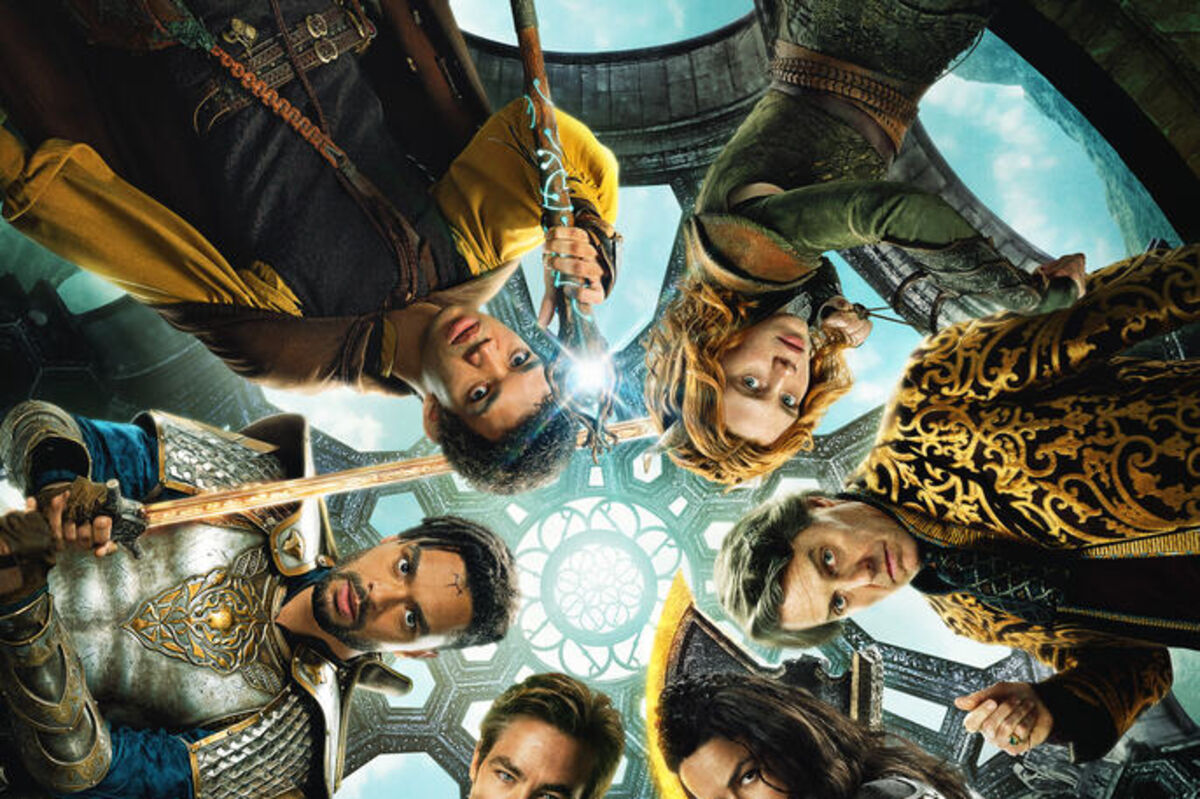In this bottom-up perspective photograph, a diverse group comprising approximately eight people is captured looking down at the camera. Among them, two are women and the remaining individuals are men. Each person displays an inquisitive expression, as if puzzled about the reason behind the photograph or seizing the chance to express a bit of their personality. Several of them adopt power stances, conveying a sense of confidence and assertiveness. The unique vantage point and the varied reactions of the subjects combine to create an intriguing and dynamic image.